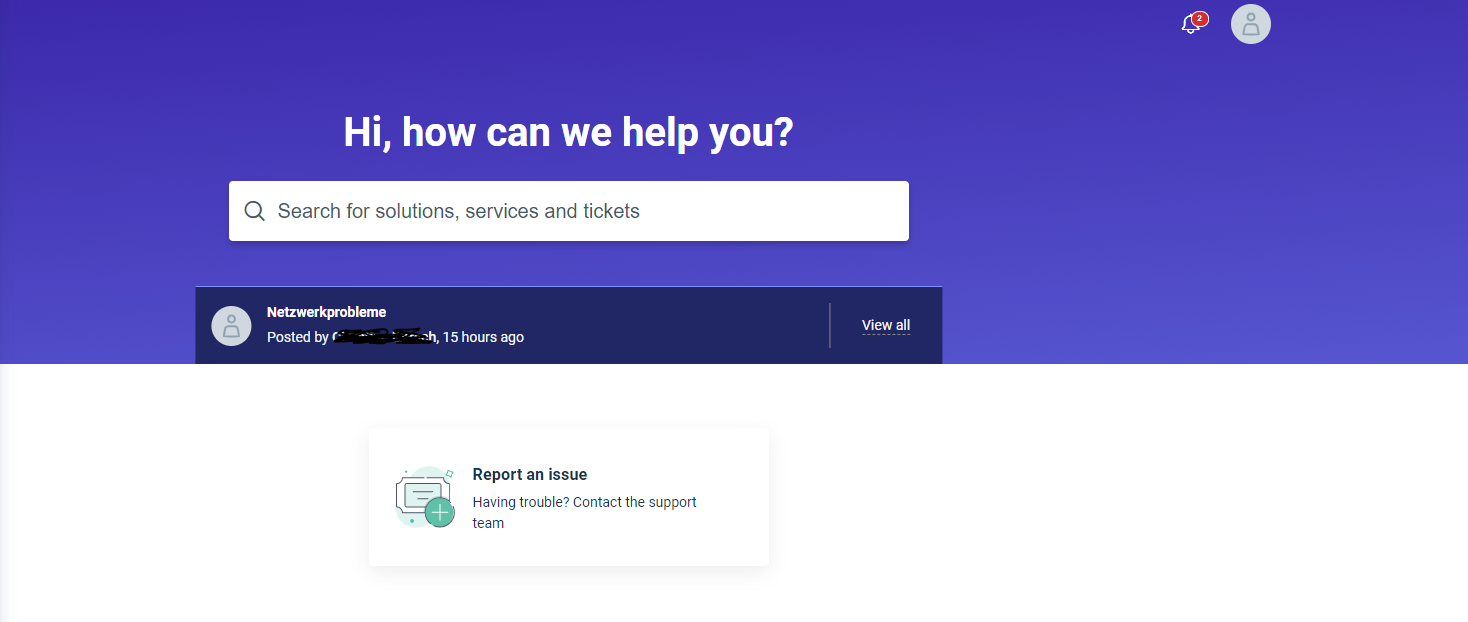Screenshot of a webpage featuring a blue banner with white text. At the top-right corner of the page, there is a circular profile button and a red notification bell indicating one new notification. The notification alert is displayed in red with a bold white font text saying, "Hi, how can I help you?". Below the banner, there is a search bar accompanied by a magnifying glass icon with placeholder text reading, "Search for solutions, services, and tickets."

Further down, a blue pop-up appears showing account information. Within this pop-up, a profile button is visible. A post regarding "Net's work problem" is mentioned, although the author’s name has been blacked out. The post was made 15 hours ago, and there is an option to "View all." At the bottom of the screen, there are several support options including, "Report an issue," "Having trouble," and "Contact the support team." A green and white button featuring a plus sign is also visible.